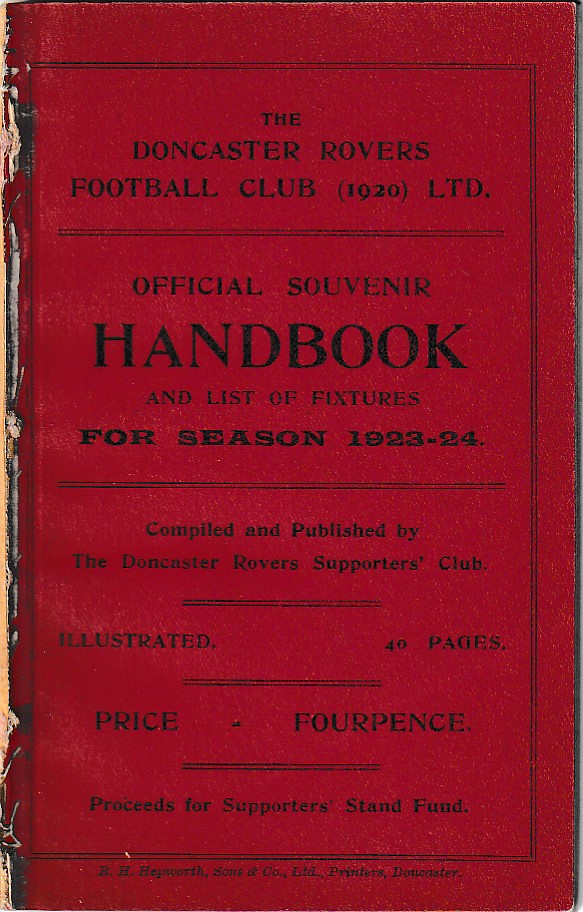The image depicts a vertically aligned rectangular cover of an exceptionally worn book. The deep, rich red cover is adorned with black printing and features a thin black border around all the text. Most notably, the spine is almost completely worn away, with visible rips and deterioration where the book opens. The text on the cover reads: "The Doncaster Rovers Football Club, 1920, Limited. Official Souvenir Handbook and List of Fixtures for Season 1923-24" centered at the top. Below this, the cover states: "Compiled and Published by the Doncaster Rovers Supporters Club," followed by "Illustrated, 40 pages." The price is listed as "4 pence," and the proceeds are designated "for the support of Stand Fund." At the very bottom, although partially illegible, it appears to say "R.H. Hepworth, Sons & Company Limited, Printers Doncaster." The prominent word "Handbook" is centered in bold, capturing attention amid the detailed historical and contextual information of this British football club memorabilia.